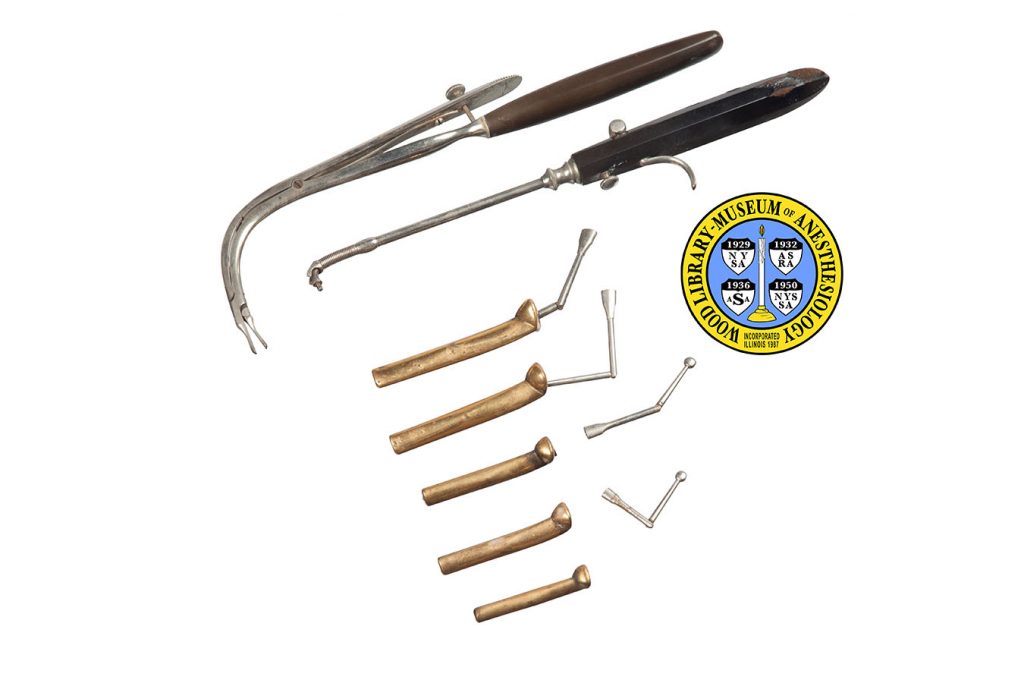This color photograph, taken from a top-down perspective, showcases a selection of medical tools, specifically used in anesthesiology. The centerpiece items are two larger tools. The first tool features a long brown wooden handle attached to a metal shaft which curves at a 90-degree angle, ending in tweezer-like adjustable pincher tips. This tool includes a screw near the handle that allows it to be held open or closed. The second tool also has a brown handle, but its metal shaft is straight and sharp, though it also curves slightly near the tip. Both tools appear to be designed for interchangeable parts, indicated by the presence of screws.

Below these primary tools, there are five smaller brass and brown-gold components that seem to be attachable tips or bits for the larger tools. These smaller pieces resemble camel feet with various burrs coming off them.

To the right of these tools lies an emblem from the Wood Library Museum of Anesthesiology. The emblem is yellow with a blue interior, featuring a central candle-like symbol surrounded by four shields bearing different dates (1929, 1932, 1936, 1950) and corresponding initials (NYSA, ASRA, ASA, NYSSA). At the bottom, it reads "Incorporated Illinois, 1967," albeit with some difficulty in reading.